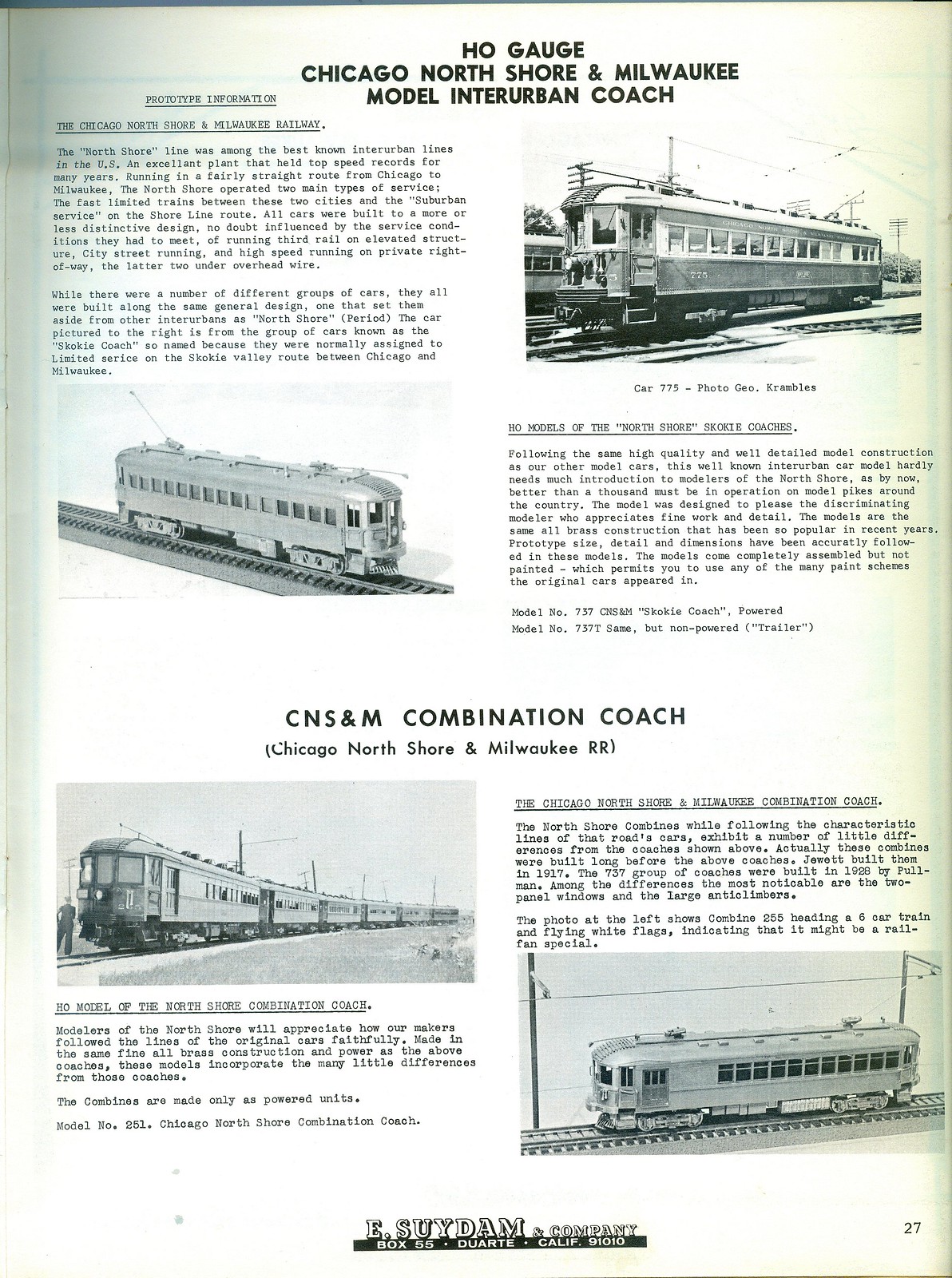This vertically aligned, black-and-white image captures a detailed page numbered 27 from a booklet or magazine. The title centered at the top of the page reads, "Ho Gage Chicago North Shore and Milwaukee Model Interurban Coach." The left half of the page features several left-aligned paragraphs of text describing the Chicago North Shore and Milwaukee Railway. Adjacent to this text on the right, there's a picture of a train labeled "Car 775 Photo Geo Crambly Crambles."

On the bottom half of the page, a centered heading declares "CNS&M Combination Coach (Chicago North Shore and Milwaukee RR)." This section includes additional text on the left side, while to the right, there's another left-aligned paragraph beneath a photograph of a model train. The image of the train shows it on a slightly curved track, enhancing its realistic depiction. At the lower right corner, another picture of a train accompanies a short paragraph. The text at the bottom mentions "East So Suit Swedam and Company Box 55, Dwart California 90910."

This image provides a comprehensive description of the model trains and coaches associated with the Chicago North Shore and Milwaukee Railway, enriched with historical photographs and detailed captions.